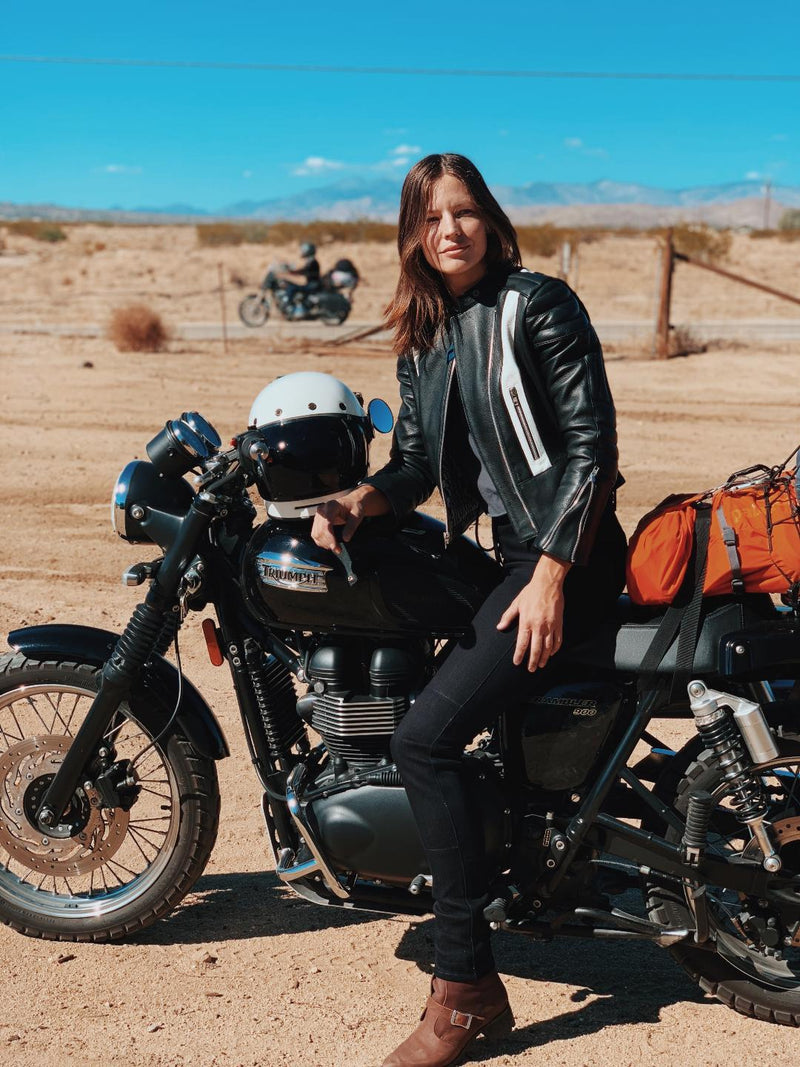The image captures a young Caucasian woman with shoulder-length brown hair seated on a black motorcycle, which is facing slightly away to the left. She is turning her head towards the camera. The motorcycle, set on sandy ground, features a silver emblem with indistinct writing on the front, and a white helmet is placed prominently atop the vehicle. The woman is dressed in a black leather jacket, black jeans, and brown boots. Behind her on the motorcycle is a small orange bag.

The backdrop reveals a desert setting with sand and rocks underfoot, extending into the background where a road cuts across the scene. Another motorcyclist can be seen riding from right to left on this road. Beyond the road lies more sandy terrain dotted with dry, brown bushes. Further in the distance, large hills rise beneath a clear, bright blue sky. A single power line traverses the upper part of the image, completing this serene and expansive desert landscape.